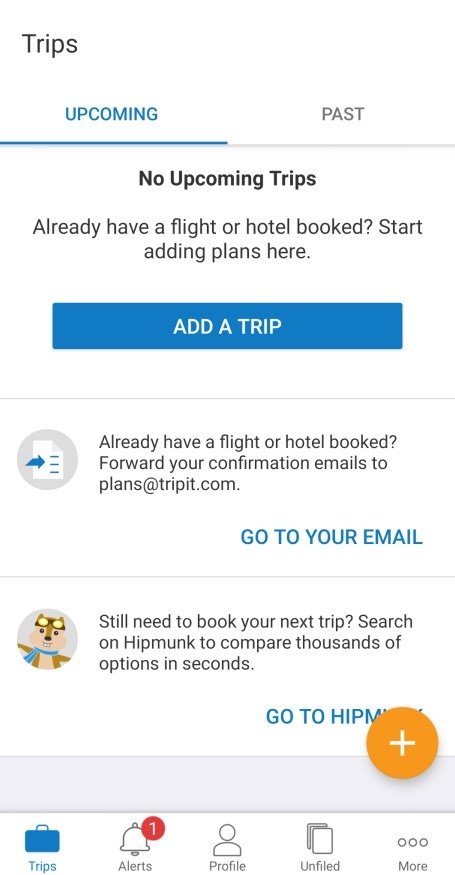The image displays an application interface titled "Trips" from TripIt. In the upper left corner, there are two tabs: "Upcoming" and "Past." The "Upcoming" tab is highlighted in blue, indicating it is currently selected, while the "Past" tab is greyed out. Below the "Upcoming" tab, there's a message in black text stating, "No upcoming trips," accompanied by a prompt that reads, "Already have a flight or hotel booked? Start adding plans here." Beneath this prompt is a blue button labeled "Add a Trip" in white text.

A fine grey line runs horizontally across the screen, below which is a grey circular icon featuring a sheet of paper with a blue arrow pointing to it. To the right of this icon, text instructs users with, "Already have a flight or hotel booked? Forward your confirmation emails to plans@tripit.com." Below this, there's a blue link labeled "Go to your email."

Another grey line continues below this section, followed by another grey circular icon, this time with the image of a squirrel. Adjacent to this icon, text suggests, "Still need to book your next trip? Search on Hipmunk to compare thousands of options in seconds," along with a blue link saying "Go to Hipmunk." Notably, an orange circle with a white "X" overlays part of the word "munk."

At the bottom of the screen, there is a grey border containing a series of navigation icons: "Trips," "Alerts," "Profile," "Unfiled," and "More." The "Alerts" icon has a small red circle with the number "1," indicating a pending notification.